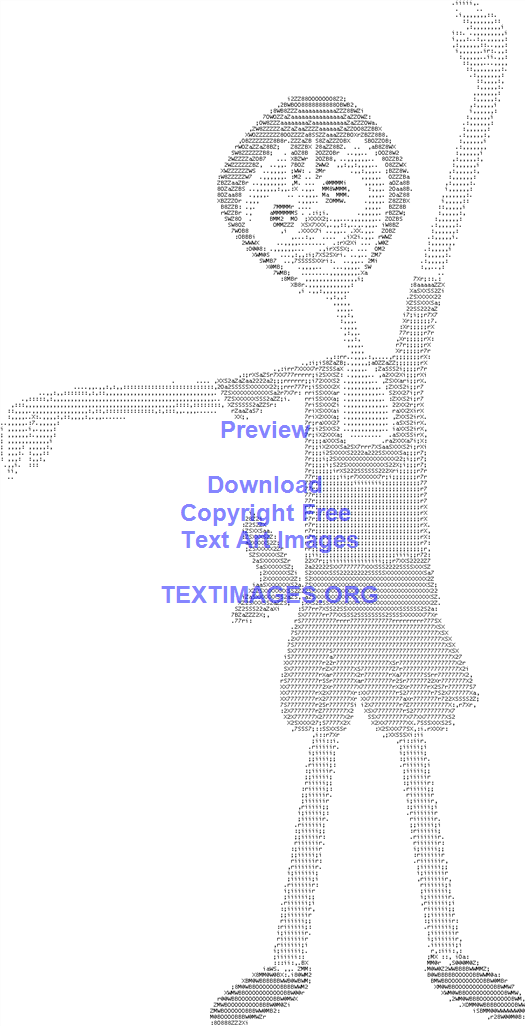The image features a pixelated, cartoon-like digital design of a little girl with short hair and big, googly eyes. She stands with one arm straight up in the air and the other extended out to the side, as though performing a dance. The girl is dressed in a short little dress and shoes, presented in black and white. Overlaying the image is a collection of text in light blue and purple that reads: "Preview, download, copyright free, text art images," with "textimages.org" at the bottom. The overall effect is whimsical and engaging, creating a playful and artistic representation.